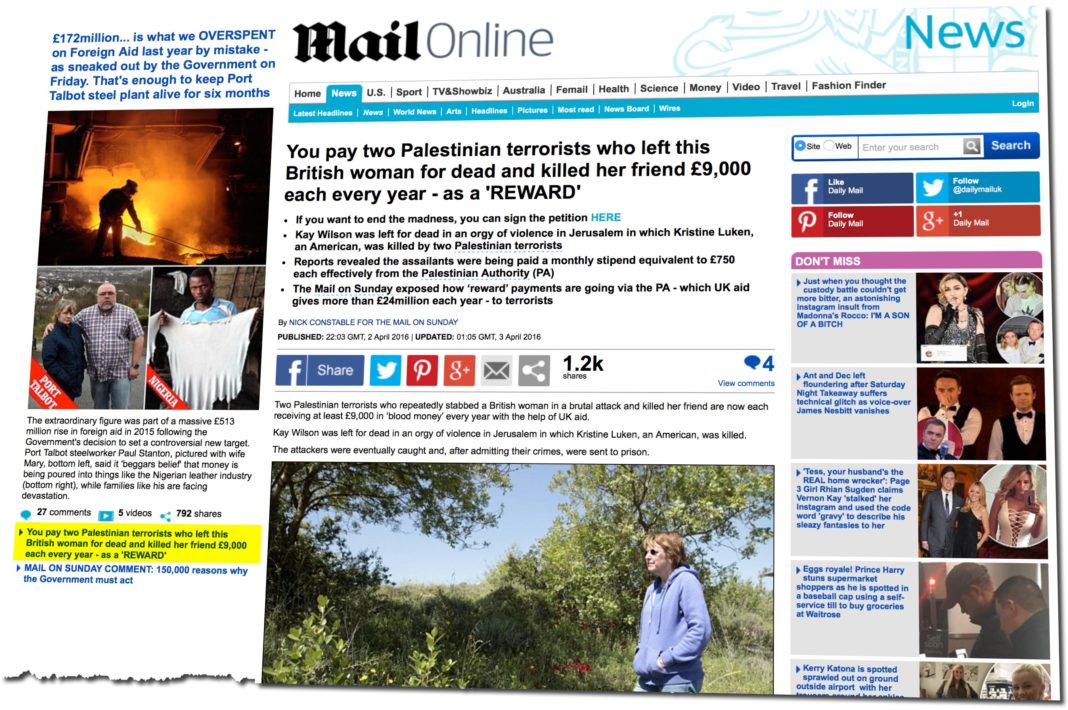This image depicts a diagonally angled photograph of the front page of the Daily Mail Online. The image is tilted upward to the right, creating a slightly skewed perspective. The bottom left corner of the page appears torn, with jagged paper edges visible. In contrast, the bottom center and right portions exhibit a faint gray shading, suggesting a fold in the paper. This shading continues up the right side, giving the impression that this section of the page is slightly elevated.

The background of the front page is white, and on the left side, there is a distinct panel containing an article. This article, at its bottom, displays engagement metrics: 37 comments, 6 videos, and 792 shares. Below these metrics, a key point from the article is highlighted in yellow. To the right of this left-side panel, the Mail Online logo is prominently featured. On the far right side of the page, the word "News" is presented in large, bold blue letters.

Just below the Mail Online logo, a row of categories spans horizontally across the page, with "News" being the selected category. The main body of the front page features a prominent story accompanied by a large photograph situated towards the bottom center of the page. This visual arrangement draws attention to the central story highlighted in this edition of the Daily Mail Online.